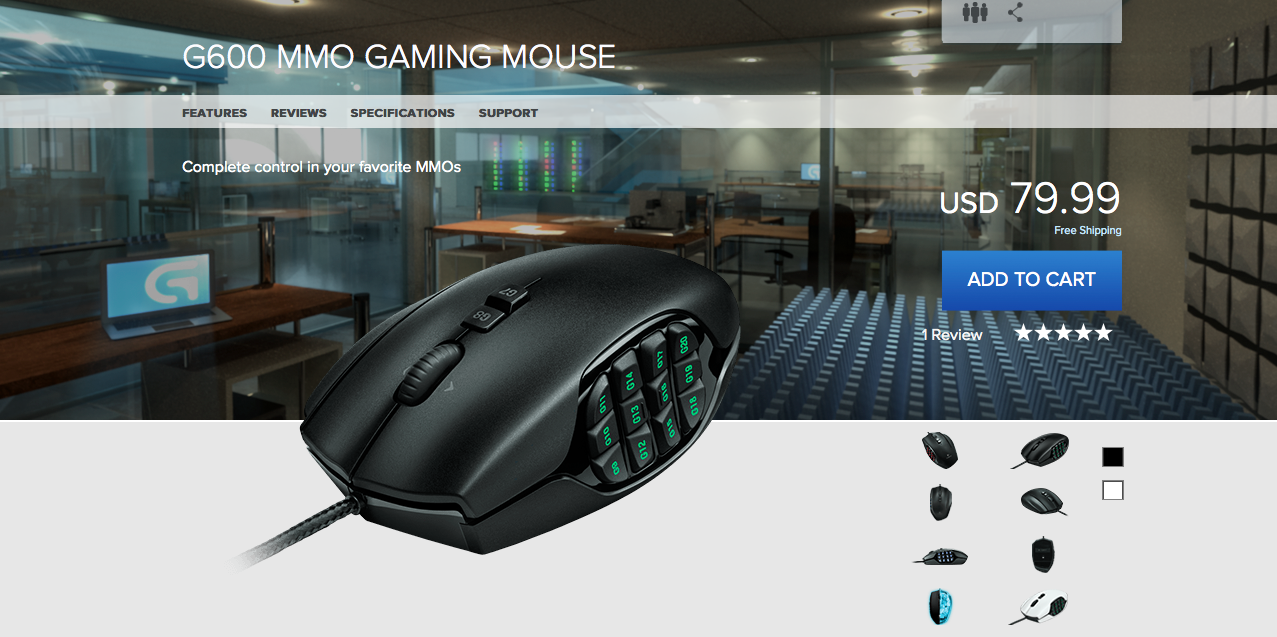This screenshot captures a promotional webpage for the G600MMO Gaming Mouse. Dominating the top two-thirds of the screen is a photograph of a modern office space. The office is furnished with blue and white carpeting and features a distinctive glass block wall to the right. The back wall is entirely made of glass, providing a glimpse into another office area equipped with desks and additional glass partitions.

In the upper left corner of the image, "G600MMO Gaming Mouse" is prominently displayed in white, all-caps lettering. Directly below this title, a horizontal gray rectangle spans the screen, containing black text for navigation options: Features, Reviews, Specifications, and Support.

Three lines below this navigation bar, white text reads, "Compare, Control, and your favorite MMOs." Slightly left of center, there is a detailed, close-up image of the black G600MMO Gaming Mouse. This corded mouse has a visible cord extending downwards to the left. It features a roller bar and multiple buttons on its top surface. The side of the mouse is equipped with an array of twelve black-numbered keys, arranged in three rows of four, highlighted with green text.

Above and to the right of the mouse image, the price is displayed in white as "USD $7.99." Directly below this price is a blue rectangular button with the text "Add to Cart" in white. At the bottom right corner of the screen, there are additional views of the G600MMO Gaming Mouse, providing different perspectives of its design and functionality.